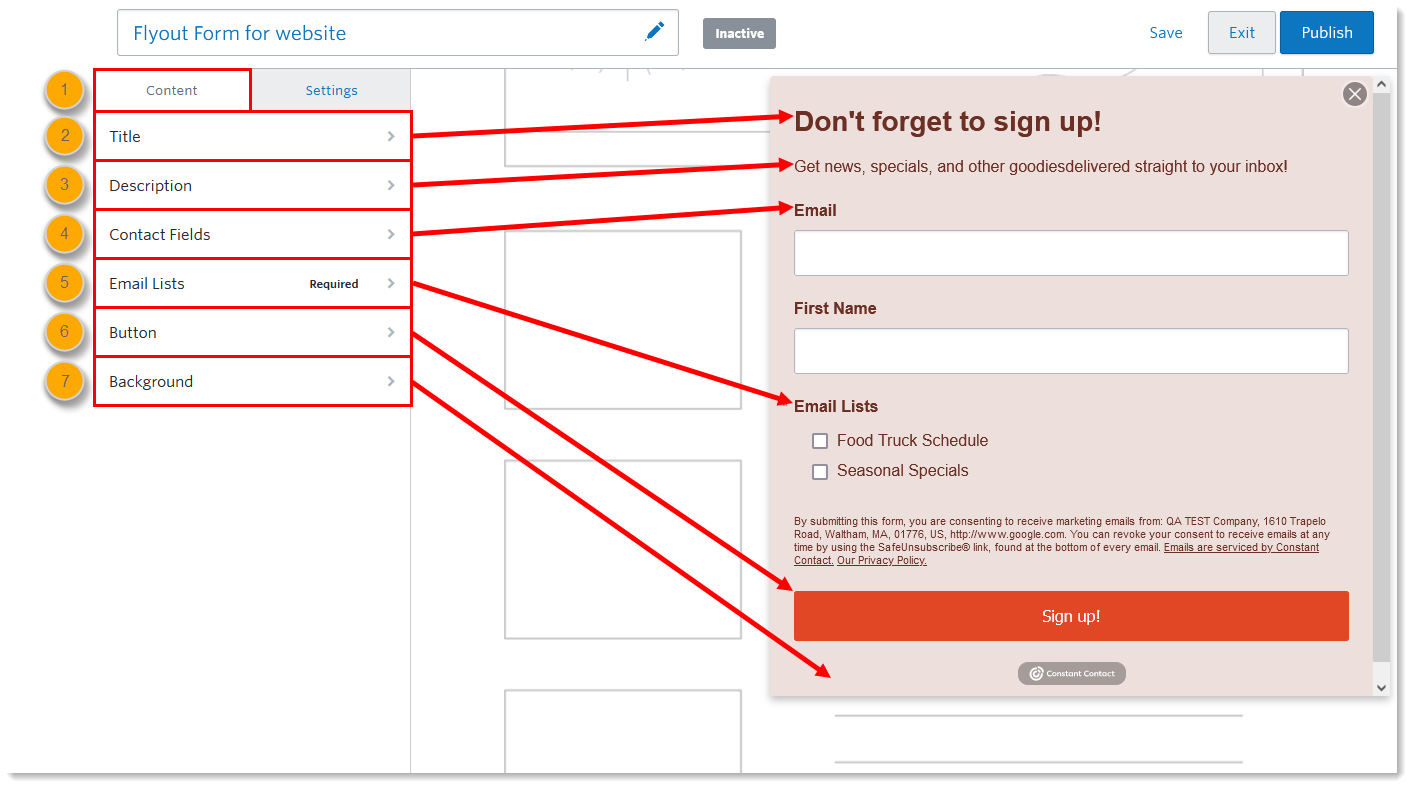The image shows a screenshot of a web page titled "Fly Out Form for Website," displayed prominently at the top left in blue text. This title is set against a white background, bordered by a light gray horizontal rectangle. Immediately to the right, in a gray box with white lettering, is the word "Inactive." On the top right corner, three buttons are visible: "Save" in blue text, an "Exit" button in blue, and a "Publish" button with a blue background.

Below this header, an item list is presented on a white background and outlined in red. Each item in this list is written in black text, contained within its own connected horizontal rectangle box. Red arrows, gradating from orange to red, extend from these list items to corresponding sections on the right side of the page.

For example, the first arrow points to the word "Title" and leads across to a black bold text reading, "Don't forget to sign up." Further down the grid, which is numbered one through seven with orange circles to the left of each grid box, is a description. Here, the red arrow points to the text: "Got news, specials, and other goods delivered straight to your inbox."

Finally, there is a red folded sign-up area prominently featured on this page, indicating a call-to-action for users to engage with. The thorough visual structure guides the viewer through the different sections and call-outs methodically.